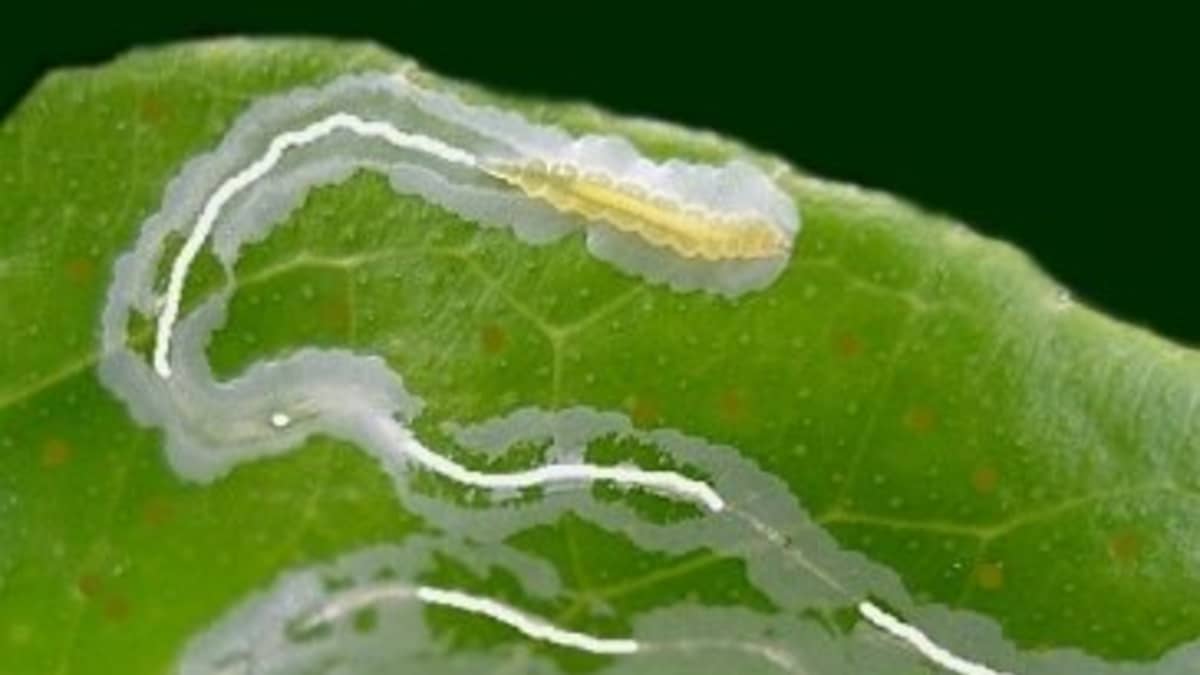This highly detailed close-up photograph showcases a lime green leaf with intricate yellow veins and speckled with small white-yellowish, larger light brown spots, and a distinctive black marking along the top, growing larger from left to right. Dominating the scene is a fascinating slime trail originating from the bottom left, meandering through various twists and turns including a loop at the top, and culminating near the middle-left portion of the leaf. This path, varying in thickness and slime coverage, features a persistent white line within it. At the heart of this scene is a transparent, clear-bodied yellow caterpillar-like larva. The larva’s elongated body is segmented with visible, clear yellow nodules and exudes white threads as it travels along the leaf, adding to the mesmerizing complexity of this nature microcosm. Against a stark black background, the contrast emphasizes the intricate details and mesmerizing journey of the larva on this vibrant leaf.